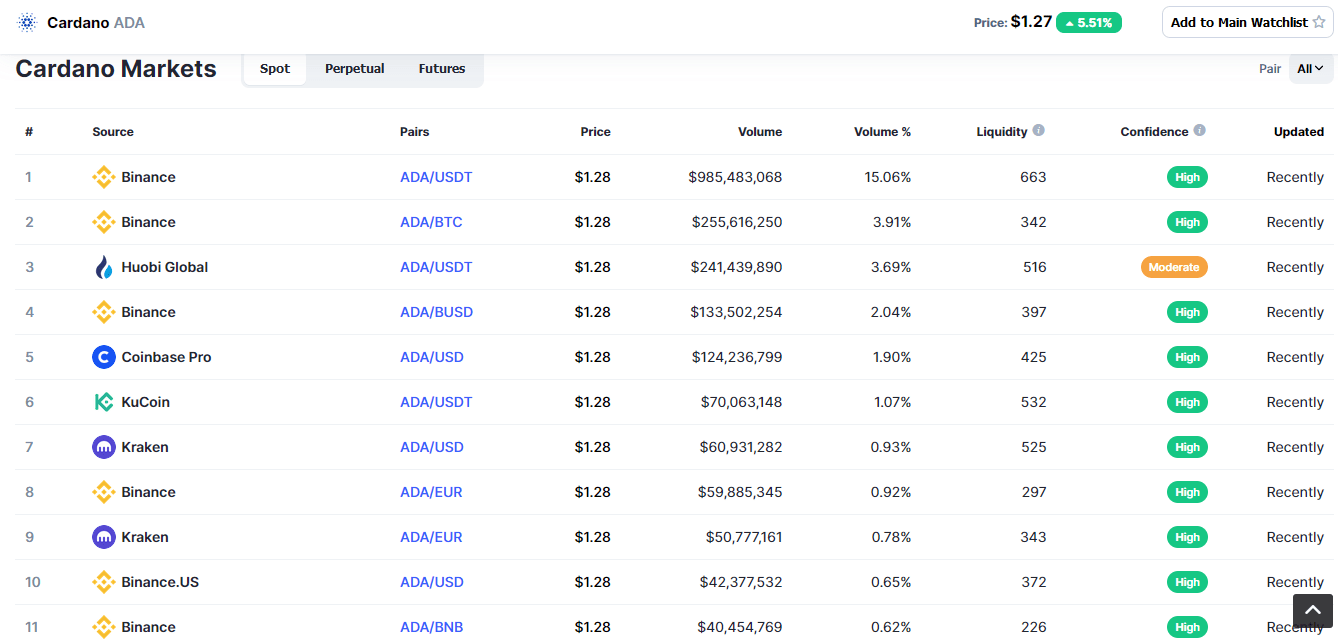Screenshot of Cardano ADA Price Data

The image displays a detailed screenshot of Cardano (ADA) price statistics against a white background. The Cardano ADA price is prominently shown as $1.27. The layout is a rectangular section that includes an option to "Add to Main Watch List" represented by a star icon. The screenshot highlights the "Cardano Markets" tab which contains various subsections such as "Spot" (highlighted in white), "Perpetual," "Futures," "Pairs," and "All".

Below these headings, there are columns labeled "#" (number), "Source," "Pairs," "Price," "Volume," "Volume %," "Liquidity," "Confidence," and "Updated." Each column contains specific data entries.

- The first entry shows the number 1, and the source is Binance. The pair is ADA/USDT, with a price of $1.28. The volume displayed is $985,483,068, representing 15.6% of the total volume. The liquidity score is 663, and the confidence level is marked as high. The update status is marked as "recently."

- Other listed items include similar attributes where high confidence is consistently noted, except for the third item. The last item listed is Binance ADA/BTC.

This detailed visualization provides comprehensive information for Cardano traders and enthusiasts, ensuring they are well-informed about market dynamics on Binance.